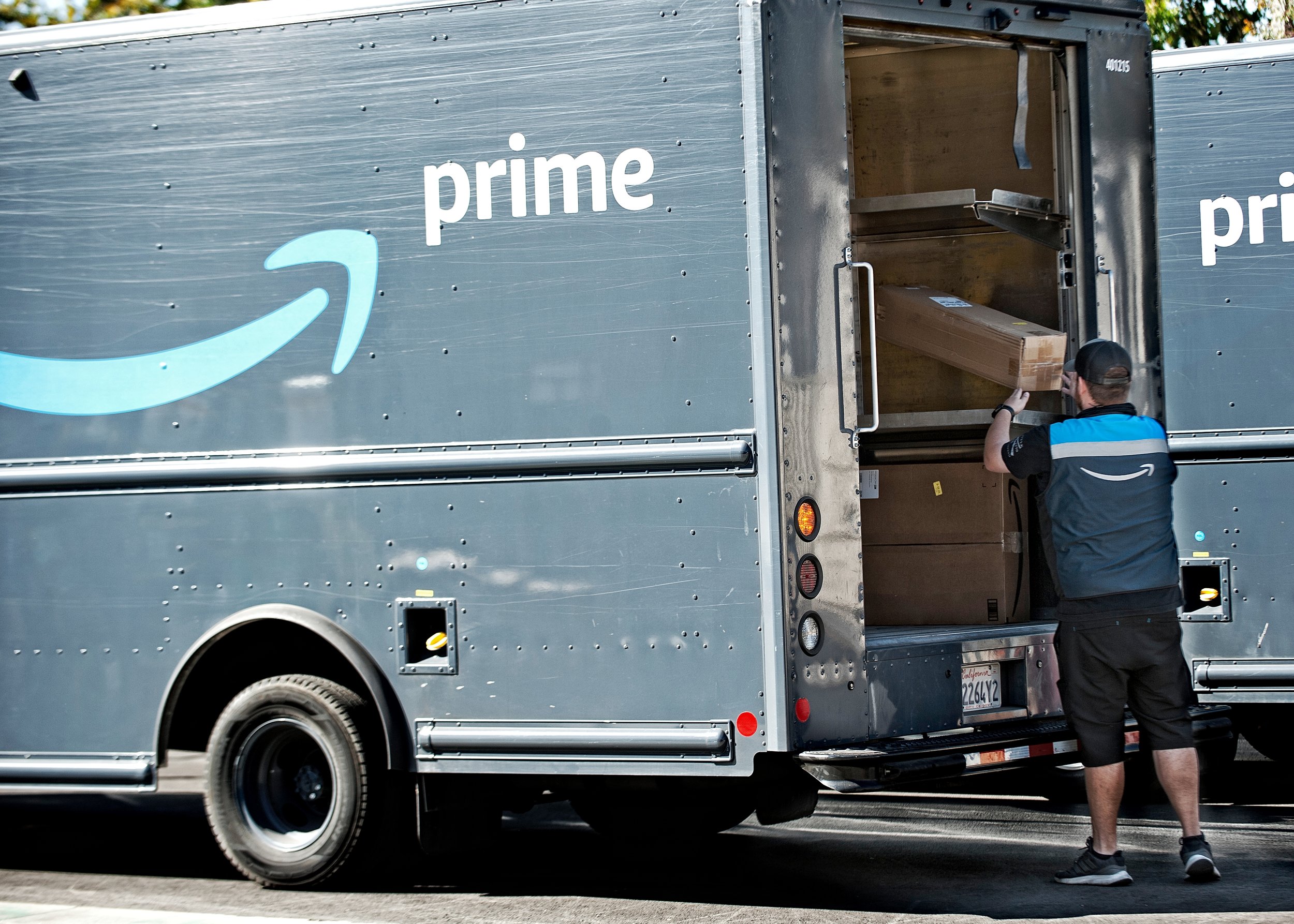In this image, the upper part features a few trees and glimpses of a light blue sky. On the right side, more trees are visible. The scene centers around a street with an Amazon Prime delivery truck in a bluish-gray color. The truck displays the iconic "Prime" logo with a swoosh arrow. The driver, positioned at the back of the truck, is equipped in a gray puffy vest adorned with the same swoosh arrow and blue and white stripes, a black cap, black watch, black tennis shoes, and black shorts. He is actively pulling a package off the truck. The vehicle's back end features distinctive yellow, red, and white lights, along with a white tag and additional red and white lights along the bottom. Adjacent to this truck is another Prime vehicle, where details like the open gas cap and small brads on the side are visible. The truck also has several white spots along the backside, including near the tail, and a small red circle towards the lower part of the side.